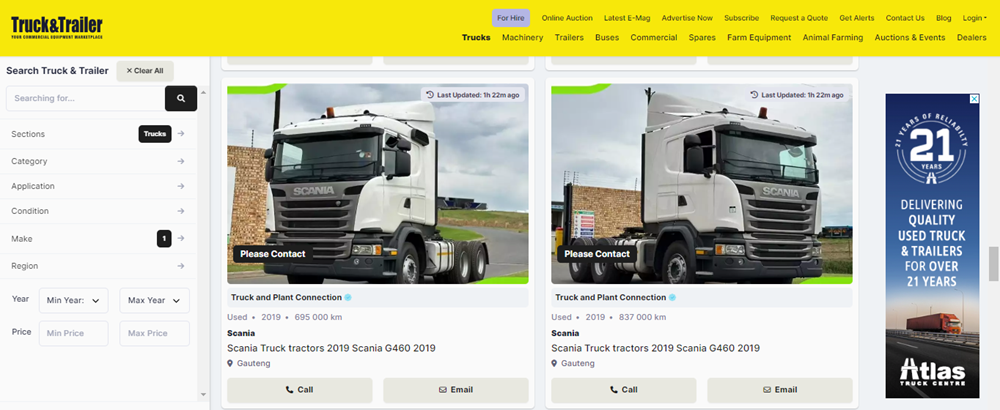This image features two Scania truck cabs parked side by side on a country road, showcased against a scenic backdrop of green grass, trees, and a sky dotted with light blue clouds. The trucks' bodies are primarily white with gray front fenders, and they prominently display the Scania brand name on their front fenders. The picture is part of a website dedicated to selling trucks and tractor trailers, indicated by a large yellow rectangle at the top of the image. This yellow banner features "Truck and Trailer" written in black and white text and includes various categories like trucks, machinery, trailers, buses, commercial, spares, farm equipment, animal farming, auctions and events, and dealers. Below the primary image, two smaller images show the truck cabs from different angles. The first cab is labeled "used 2019" with a mileage of 695,000 kilometers, while the second cab, also labeled "used 2019," indicates a mileage of 837 kilometers. The setting includes a tan brick or wooden wall in the background, enhancing the rural ambiance of the scene.